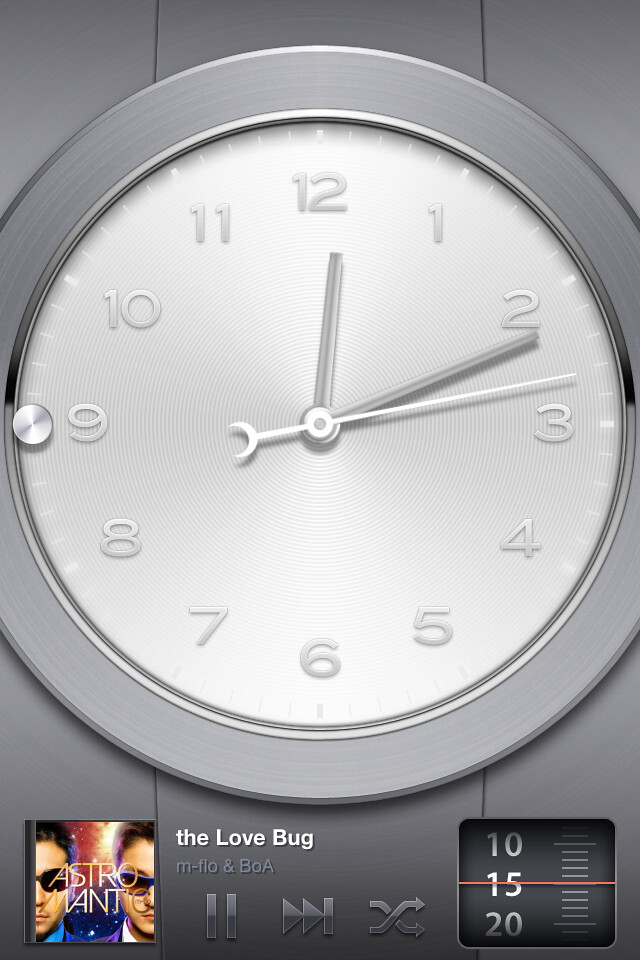The image depicts a silver circular clock against a dark gray background. The clock features a textured silver face with intricate circular patterns, silver numbers marking the hours, and three distinct hands: a short silver hour hand, a long silver minute hand, and a thin white second hand with a crescent moon at its tip. On the clock's casing, at the number 9 position, there is a small silver dial. 

Additionally, at the bottom of the clock face, there is a square album cover featuring two men wearing sunglasses, with the title "Astromantic" displayed in white letters. The background of the album cover resembles a starry sky with shades of blue, purple, orange, and yellow. Next to the album cover, the text reads "The Love Bug" by M-Flo and B-O-A. Below the cover, there are music player control buttons including play/pause, skip, and repeat. On the right-hand side is a gauge with a black background, white numbers, and an orange marker, displaying values at 10, 15, and 20, intersected by red stripes. The entire scene gives a sense of a phone or digital device interface.